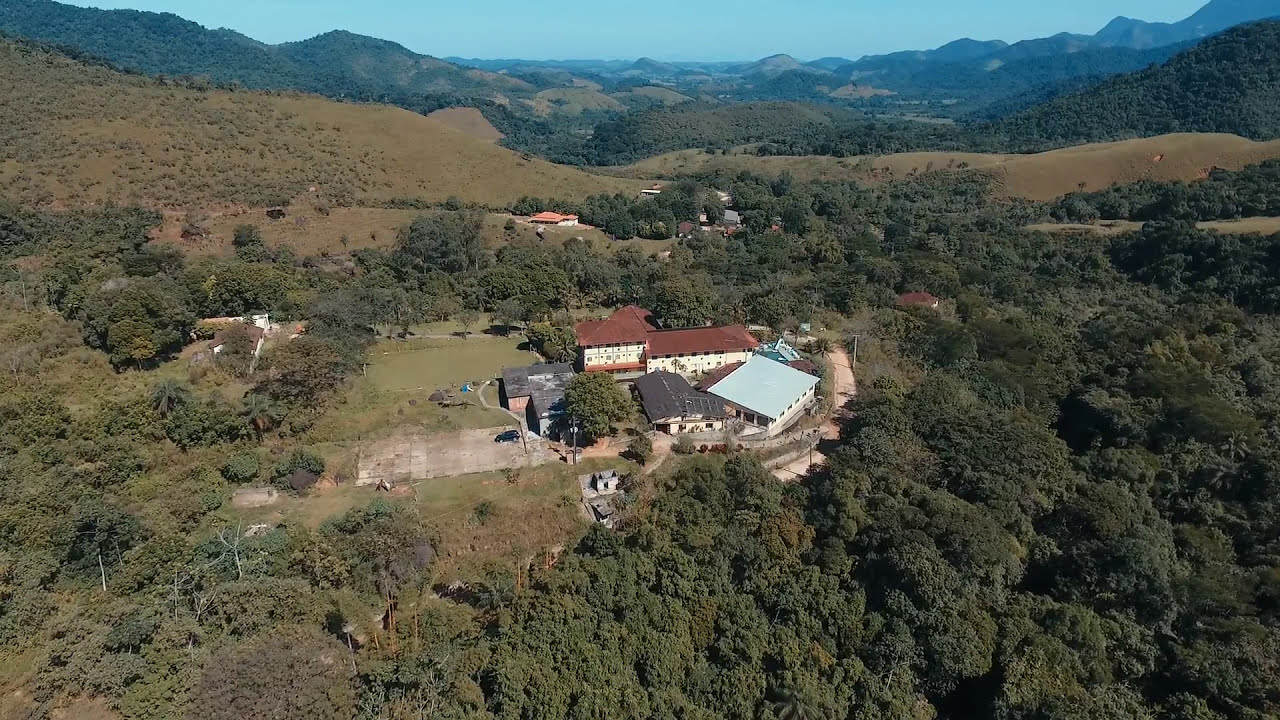This image is an aerial photograph capturing a serene and expansive landscape. At the center, there's a cluster of buildings nestled at what appears to be a private property or possibly a small school campus, set within a picturesque valley at the base of a mountainous range. The main structure is a large building with a red roof, while other shorter buildings feature varying roof colors, including brown, black, and blue. These buildings are surrounded by a clearing among lush, dense trees and interconnected by a dirt road that curves around the bottom right of the image. A concrete shed and an SUV parked in a small lot are also visible. The scene is framed by rolling green hills that ascend into jagged mountains in the distance, all under a clear, sunny blue sky, accentuated by vibrant grass and abundant natural greenery.